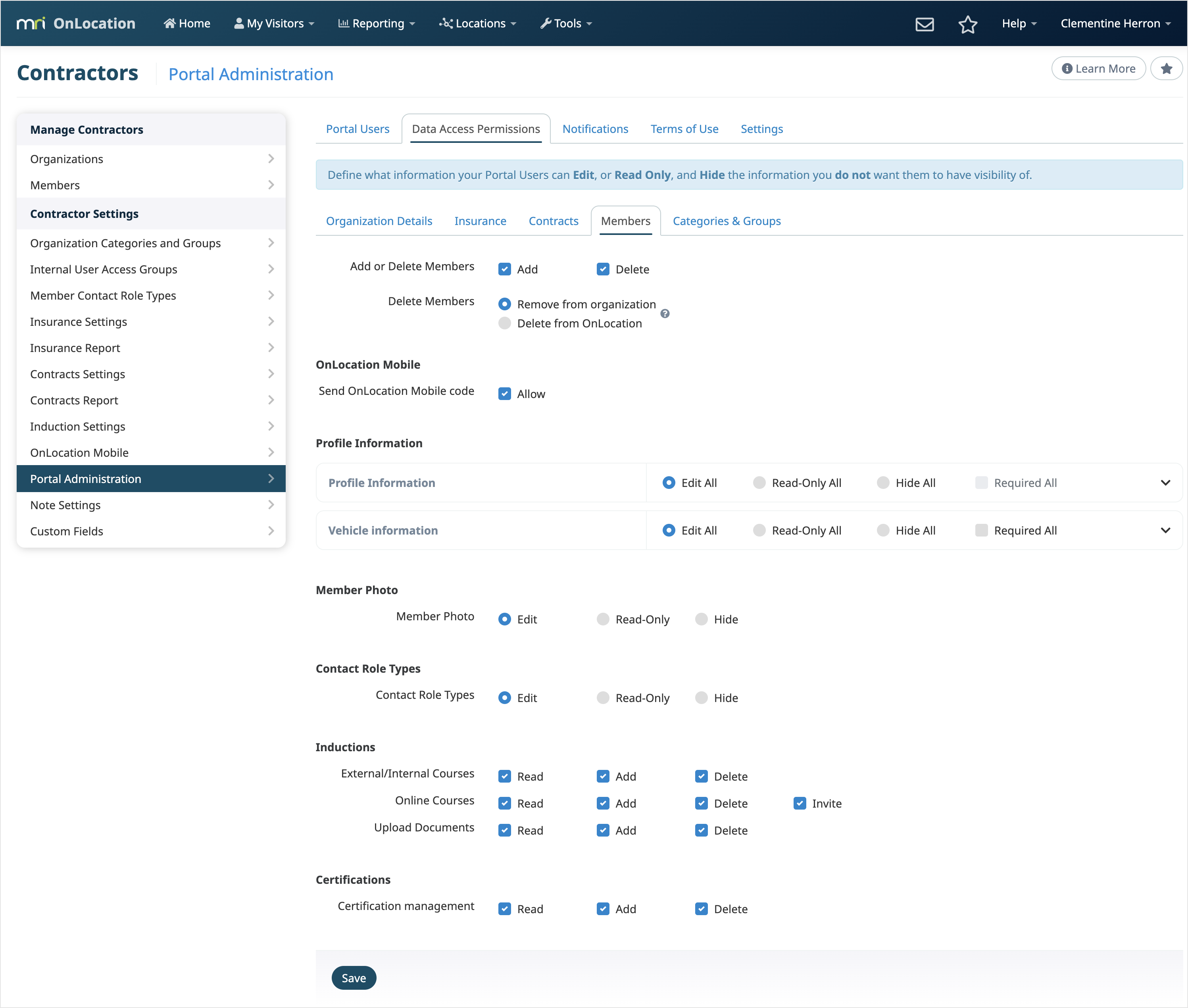This detailed desktop screenshot captures the user interface of the website "MI Contractors on Location," specifically showcasing the portal used for managing contractors. The left sidebar features an array of menu options for managing contractors, including categories for organizations, members, settings, and various administrative functions. Users can organize contractors by different criteria such as access levels, contract fee types, earnings, tests, and report settings, enabling a comprehensive overview of their data.

At the top center of the page, there is a navigation bar with several tabs. The currently selected tab is "User Access Permission," which provides an interface for controlling and viewing the access levels of different members. This page allows the administrator to view and edit member profiles, including changing profile images and adjusting various data parameters and posting permissions. This screenshot highlights the robust management capabilities of the MI Contractors on Location portal, designed to streamline contractor administration and ensure effective oversight of financial and operational metrics.